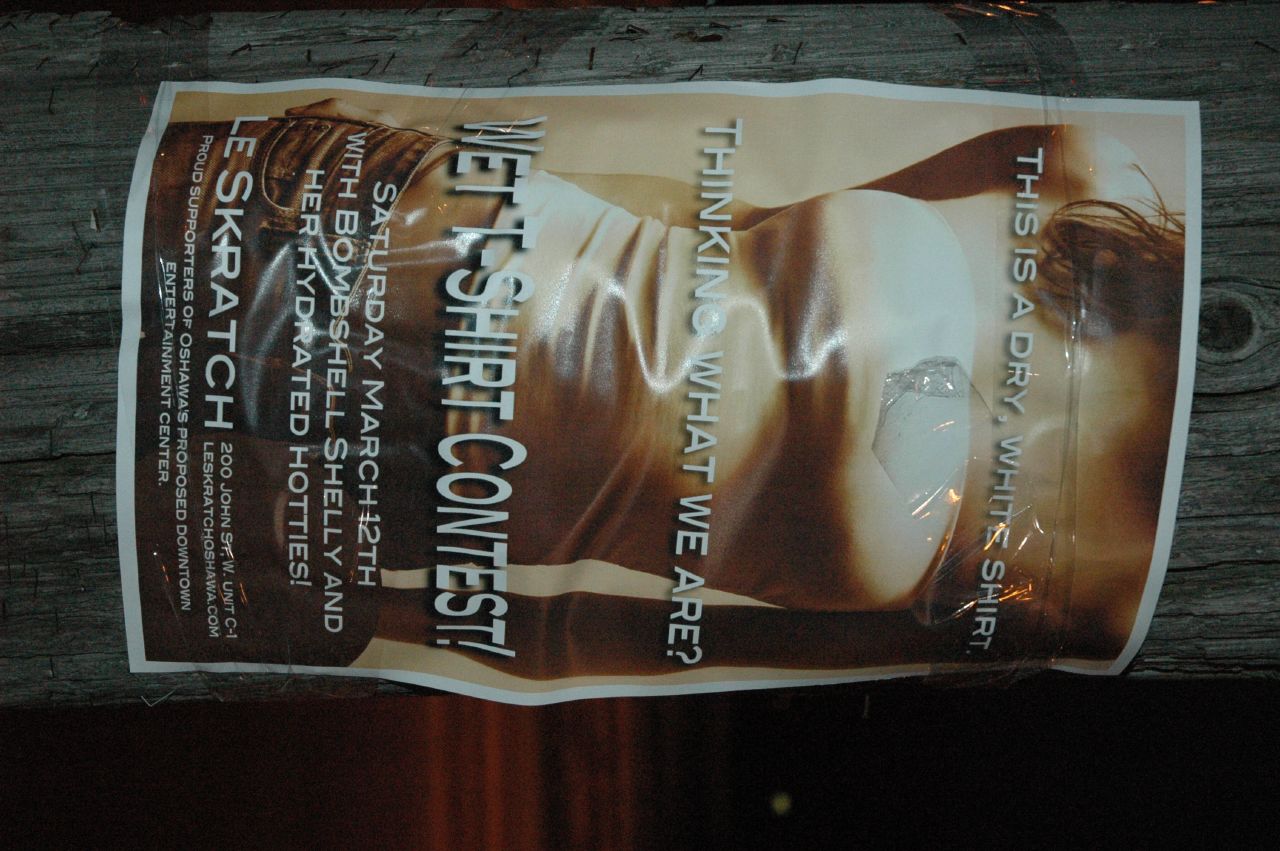The nighttime image captures a poster taped with transparent tape to a wooden telephone pole. The event advertisement features a sepia-toned photograph of a headless woman dressed in a white halter top and very short shorts, with her belly exposed. The poster showcases prominent white text, starting at the top with, "This is a dry white shirt." Below this, in the middle section, it reads, "Thinking what we are." Further down, it announces, "Wet T-shirt Contest, Saturday, March 12th with Bombshell Shelly and her Hydrated Hotties." At the bottom, it provides details: "LaScratch, 200 John Street, West Unit C1, LaScratchOshawa.com," followed by a note, "Proud supporters of Oshawa's proposed downtown entertainment center." The poster appears slightly crumpled, emphasizing its casual, gritty aesthetic.